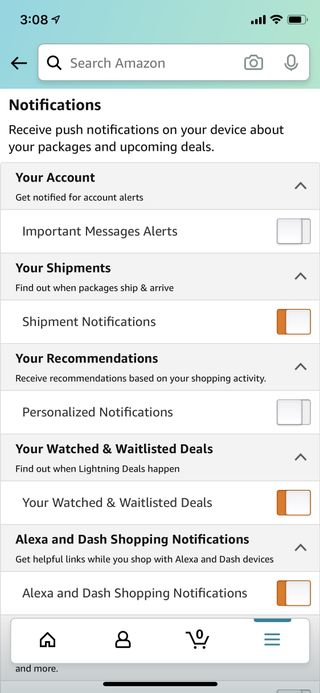The screenshot captures an Amazon interface displayed on a smartphone. At the very top, a teal navigation bar indicates a 3:08 PM timestamp, a signal strength symbol with four bars, and a battery icon showing approximately 75-80% charge. Below this, a gray search bar features options to search Amazon, accompanied by icons for a camera and a microphone.

Next, on a white background, the bold header "Notifications" highlights the section. Immediately underneath, an explanation reads, "Receive push notifications on your device about your packages and upcoming deals," suggesting the user is currently on Amazon's notification management page. 

A subsequent gray bar labeled "Your Account" is expanded, revealing a white bar underneath with the text "Important Message Alerts," which currently indicates no alerts. Following this, another gray bar titled "Your Shipments" expands to display a progress bar in a white section, showing ongoing shipment notifications.

Continuing down, a gray bar labeled "Your Recommendations" is present but currently empty. Beneath it, a gray bar titled "Your Watched and Waitlisted Deals" shows a few ongoing deals of interest. Finally, another gray bar titled "Alexa and Dash Shopping Notifications" indicates a few minor notifications, though nothing of significant importance is detailed.

Overall, the image is a comprehensive snapshot of the Amazon notification settings and account overview on a mobile device.